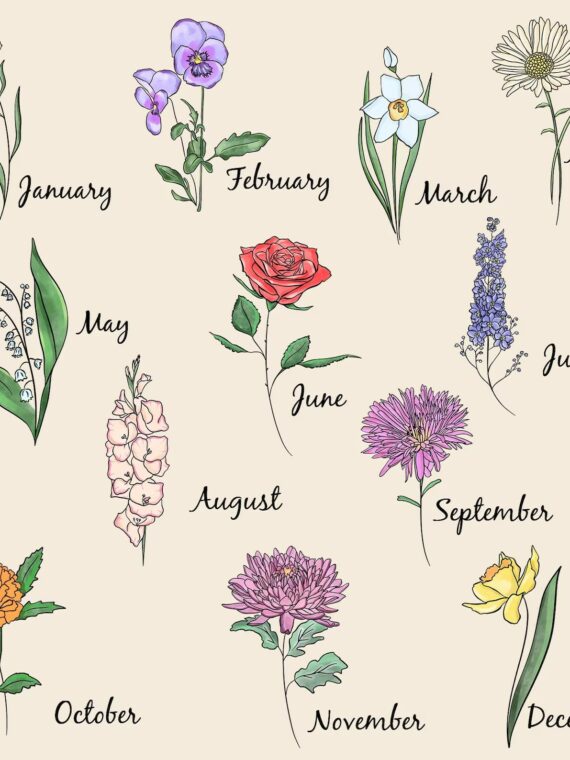The image illustrates a collection of twelve flowers, each representing a different month of the year, displayed on a pink background poster with the months written in a rustic black cursive script. Starting from the top left with January and ending at the bottom right with December, the flowers are laid out side by side. January features a tall-stemmed flower with sharp, thin leaves. February showcases a purple flower with circular petals and spiky leaves. March presents a white flower with six petals and long leaves. April has a dandelion-like flower. May’s stem is adorned with small white flowers. June depicts a vivid red rose. July displays blue bonnets. August has pink flowers. September features thin, purple-pink petals. October shows an orange flower. November resembles September's flower but with more upward-curved petals, and December concludes with a yellow flower. Each flower is vividly colored, varying from pink, purple, red, to yellow, creating a harmonious and detailed floral calendar.